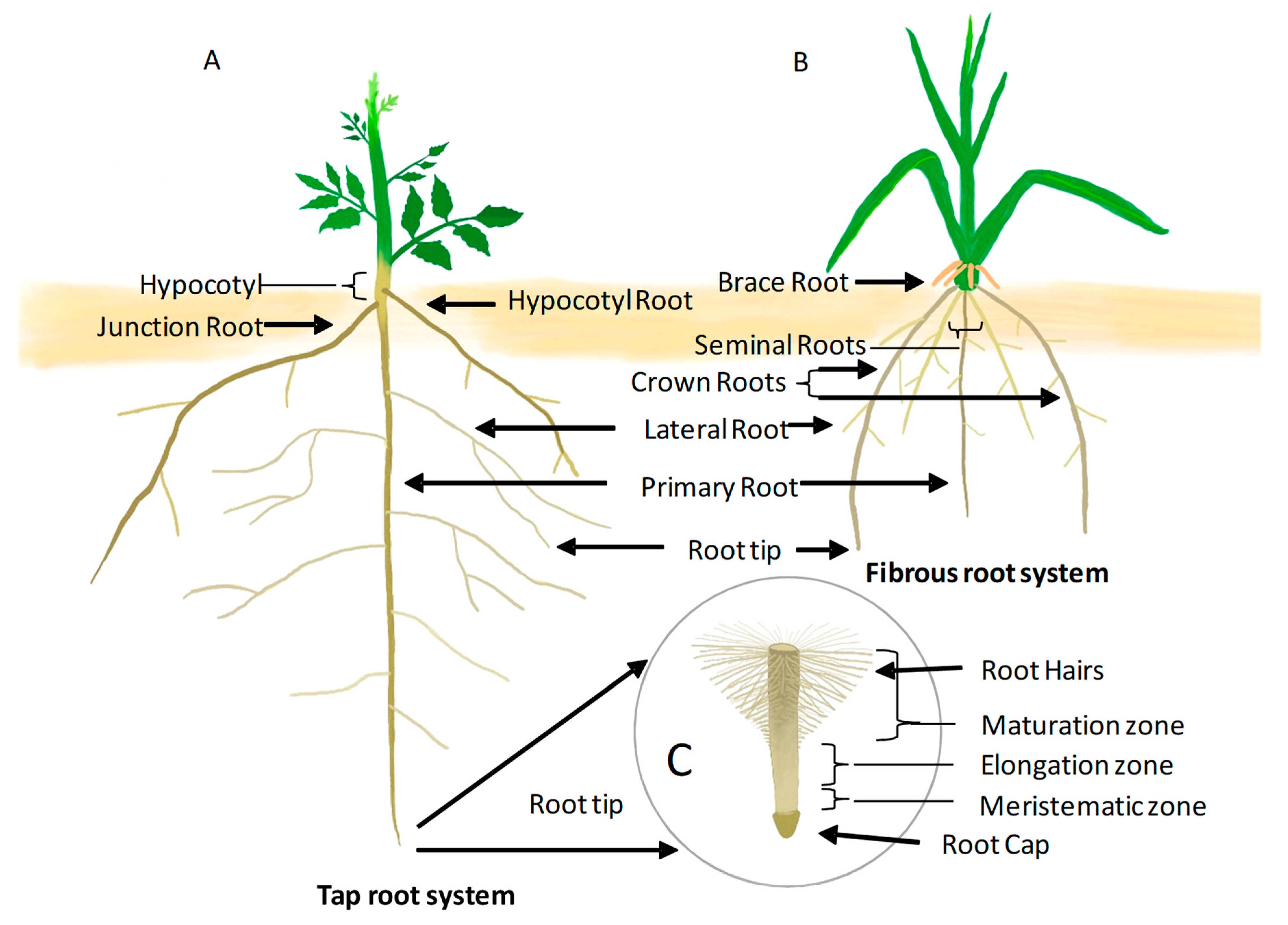This detailed scientific infographic compares the root structures of two plants labeled A and B, resembling cilantro and green onions respectively. Plant A, depicted with a short stem and four to five small branches each with five leaves, features an intricate root system that extends three times longer than the stem. This root system is detailed with labels such as hypocotyl, junction root, lateral roots, primary roots, and a taproot system, including sections like the maturation zone, elongation zone, meristematic zone, root cap, and root hairs. Plant B, in contrast, shows a leafier appearance with thin green leaves emerging from a central stalk and a different root structure labeled with brace roots, seminal roots, crown roots, lateral roots, and a root tip. Additionally, a smaller circle labeled diagram C further exemplifies a fibrous root system, illustrating components like the root hairs, maturation zone, elongation zone, meristematic zone, and taproot system. This basic yet thorough illustration effectively highlights and labels the various parts and zones of these root systems for educational purposes.